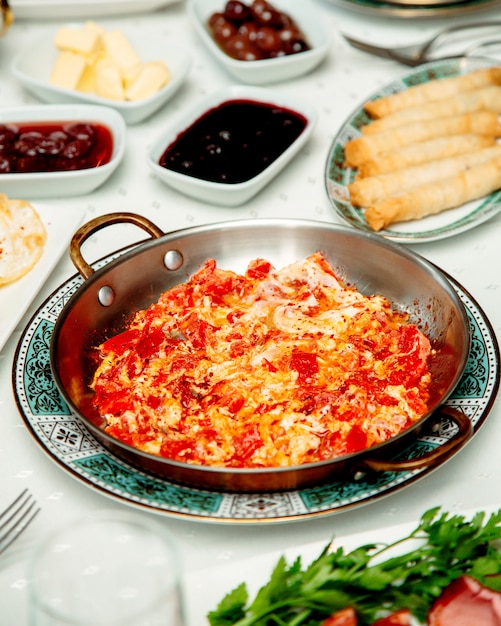The image captures a richly set dinner table featuring an array of dishes. Central to the photograph is a decorative plate showcasing alternating teal and white squares accented with ornate black filigree designs. Placed atop this plate is a shallow metal pan with copper handles on either side, containing a red and yellow dish, possibly some sort of meat or heavily spiced vegetable mixture. The dish has hints of red, orange, and white, contributing to its vibrant appearance.

In the foreground, slightly out of focus, lies a glass, a fork, and a few sprigs of herbs, adding a touch of greenery on the bottom right. Surrounding the main dish in the background, various smaller plates and bowls are visible, though they become progressively blurred. These include trays holding jams, jellies, and cubes of butter, along with plates of canned cherries and rolled items that could be chimichangas or crepes. To the upper right of the main dish, a solitary breadstick can be spotted, adding to the assortment on the table.

The tablecloth under the setting is primarily white adorned with black patterns, complementing the intricate designs on the central plate. Overall, the photograph exhibits a well-arranged and inviting dinner table with a focus on the myriad of vibrant and detailed food items.